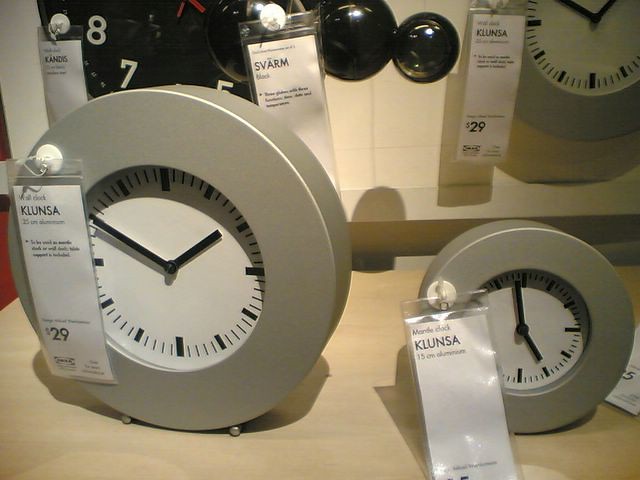The photograph captures a detailed display of various clocks within a store, identifiable by the white price tags on each item. The setting includes a light-colored table surface, which appears to have wood grains, positioned against a white wall. On this wall, there is a modern-styled clock with a silver circular frame, partially out of the image, featuring bold rectangular markers instead of numbers. Next to it, a black clock face with prominent white numbers is mounted.

In the foreground, on the table, two free-standing clocks are prominently displayed. The larger clock is on the left, approximately twice the size of the smaller one on the right. Both clocks share a similar design: a gray circular frame with a white face, marked by thicker lines in place of numerals. The lines for the 12, 3, 6, and 9 are particularly elongated, while the others are shorter but still thick. These clocks belong to the same brand, as indicated by the brand name "KLUNSA Klusner" on their tags. The larger clock is priced at $29, while the price of the smaller one is not visible. In the background on an elevated section of the table, an additional black clock with white numbers and another similar gray clock are evident, continuing the theme of the display. The modern aesthetic, price tags, and detailed clock arrangements signify a well-organized store display.